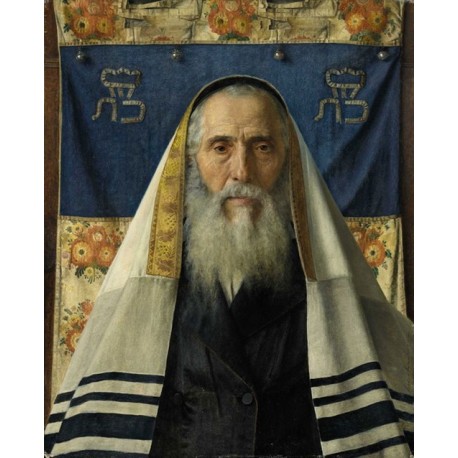This detailed painting captures a wise and venerable rabbi from the Jewish faith, depicted in full color on a rectangular, vertical canvas. The rabbi, an older gentleman with a long, gray, disheveled beard that extends several inches below his chin, has similarly gray hair peeking out from under his head covering. The head covering is a white shawl with dark gray or blue stripes at the ends and a band of gold embroidered material near the top, draping down his back. He wears a black, buttoned suit coat over a white shirt, exuding an air of solemn dignity.

The background is adorned with a dark, wooden setting, partially obscured by a floral-patterned material featuring orange and yellow flowers. Superimposed over this floral backdrop is a navy blue horizontal banner that stretches across the width of the frame, occupying about one-third of the canvas. This banner is decorated with identical Hebrew letters positioned symmetrically on each side. Despite the varying interpretations of the symbols, their presence enhances the painting's cultural depth. 

Additional elements include subtle hints of brown and black along the edges of the picture, contributing to the overall richness and texture of the scene. The entire composition radiates a realistic and detailed portrayal, adding to the gravitas and historical ambiance of the subject.